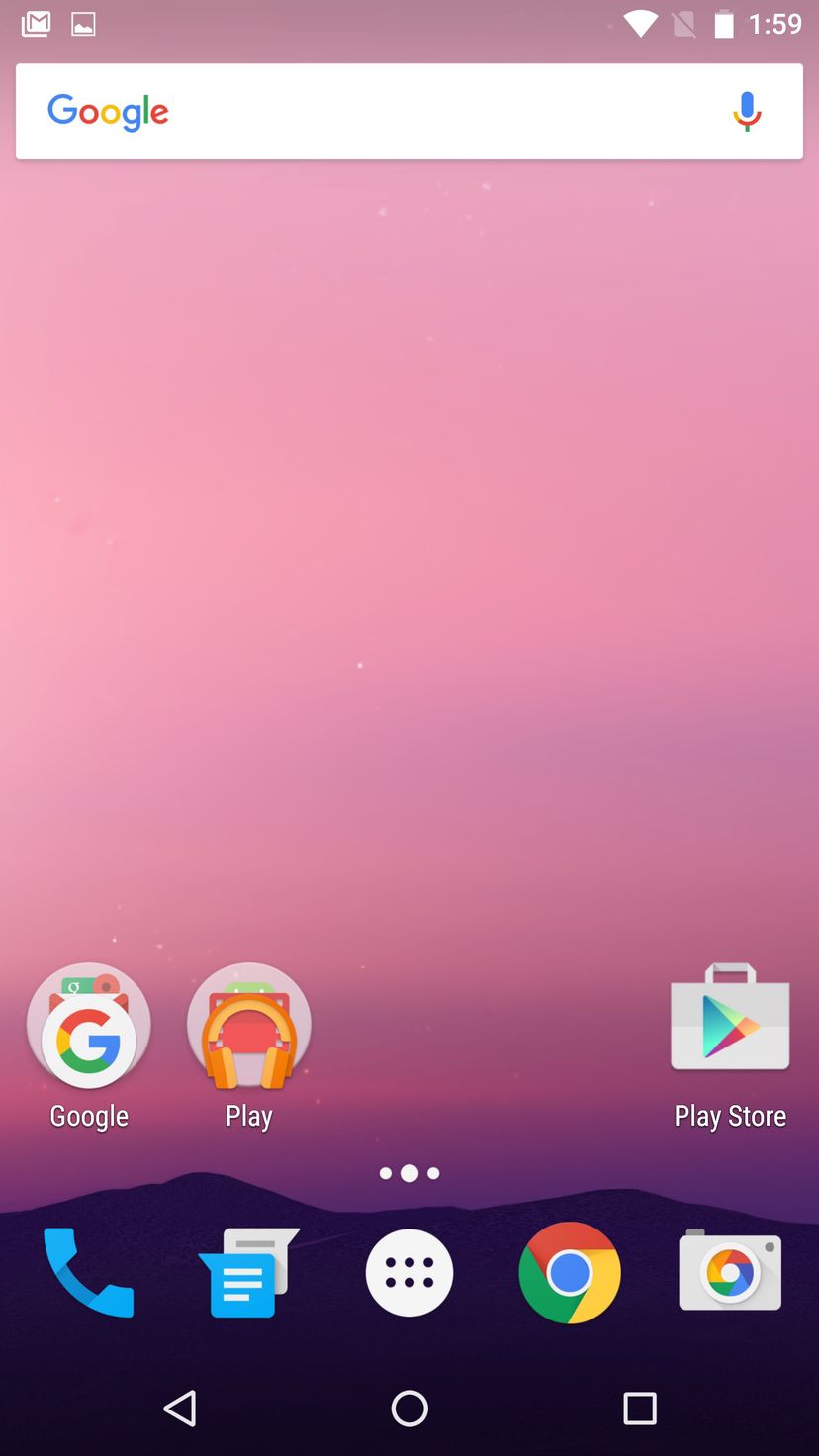The image showcases a vertical, smartphone home screen with a predominantly lavender purple background transitioning to darker shades at the bottom, resembling wavy lines that suggest mountains. In the upper left corner, there are overlapping white squares with a large lavender letter "M" in the middle. To its right, there's a white square with some white at the bottom. The typical white Wi-Fi symbol is visible on the far right, followed by a faint lavender rectangle with a line through it, and a full battery icon in white. 

The upper right corner displays the time "1:59". Below this, there is a long, thin white search bar featuring the multi-colored Google logo on the far left (a blue "G" followed by lowercase letters: a red "o", a yellow "o", a blue "g", a green "l", and a red "e"), and a microphone icon on the far right.

The main backdrop remains completely lavender purple with darker sections at the bottom. On the first row of icons, we observe from left to right:
1. A Google icon: A white circle with the Google "G" inside it, superimposing faint white circles with indistinct blue, red, and orange elements.
2. An icon labeled "Google".
3. An icon with a yellow, orange, and red half-circle at the bottom, labeled "Play".
4. A white suitcase icon with a blue triangle and shades of red, white, and orange labeled "Play Store".

Below, centered, there are three small white dots, with the middle dot slightly larger than the side dots.

Over the purple mountain imagery at the bottom of the screen, there are more icons arranged from left to right:
1. A blue telephone icon.
2. A blue text message icon with three white lines (the bottom one being shortest) and a speech bubble pointing to the upper left.
3. A partially visible white text scroll icon with a speech bubble pointing to the upper right, containing a single gray line at the top.
4. A white circle containing two rows of three black dots.
5. The Google Chrome logo.
6. A camera icon in white with elements resembling the Google Chrome logo.

Finally, at the very bottom, left to right, there are three outlined icons: a white play button, a white circle, and a white square. The interiors of these icons are purple, blending seamlessly with the background.